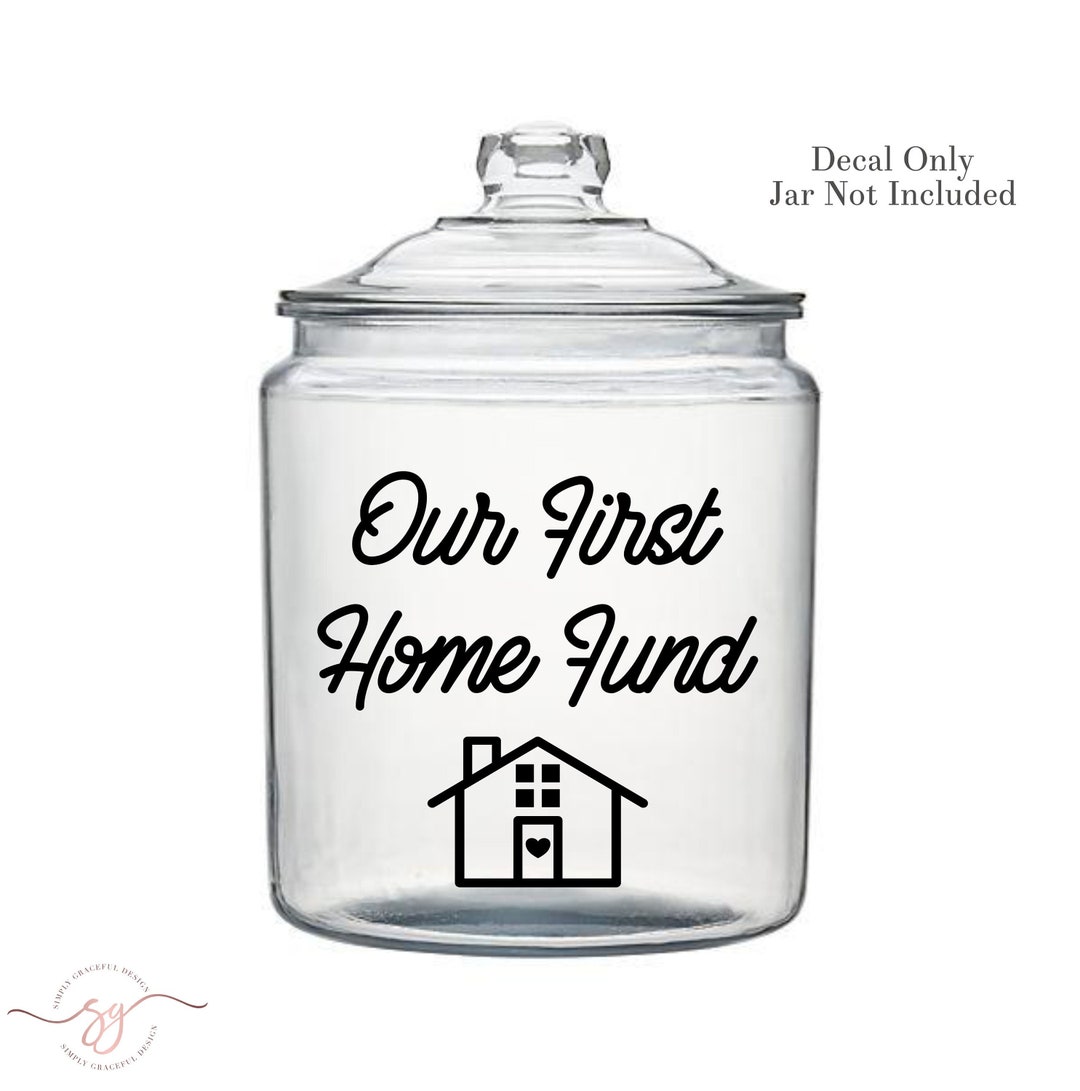The image is an advertisement for decals designed for glass jars. The main photograph displays a lidded, transparent glass jar with straight sides, resembling a cookie jar with a chunky knob on the top. The jar features a black, cursive decal that reads "Our First Home Fund," accompanied by a simple line drawing of a house with a slanted roof, a window, and a front door adorned with a heart. Notably, the upper right corner of the image includes the text "Decal only, jar not included," indicating that only the decal is for sale. The background is plain white, and in the bottom left corner, there is a small logo with the initials "SG" or "GG." The logo is circular and has a pink or red color in the middle. Overall, the ad suggests that this decal can be applied to any similar jar to create a personalized home fund container.